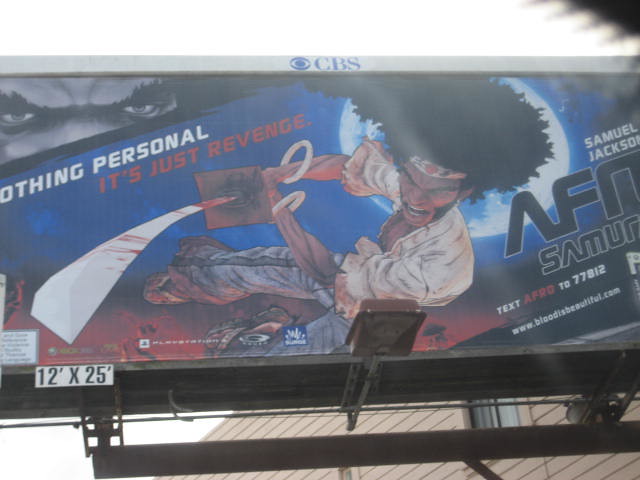The photograph showcases a large, eye-catching billboard. At the very top, the CBS logo and the letters "CBS" are prominently displayed. The main message on the billboard reads "Nothing personal. It's just revenge,” with the text aligned on the left-hand side.

To the right, the name Samuel L. Jackson is prominently featured in a highly stylized, futuristic font, along with the words "AF Samurai," indicating a probable connection to a character or series. The billboard encourages viewers to text "AFRO" to 77812 for more information. Below this call to action, in smaller lettering, is the website address "www.bloodisbeautiful.com."

The central part of the billboard is dominated by a striking cartoon figure of a black man with a large afro and a headband, resembling a ninja headband adorned with a Japanese sun symbol. He is depicted wearing an open white shirt, exposing his forearms which are accessorized with white bracelets. In his hands, he holds a large curved katana stained with blood, adding a sense of action and intensity to the image. His attire is completed by bell-bottom pants with stripes down the sides and traditional Japanese wooden sandals, known as geta, which elevate the overall samurai aesthetic.

The bottom frame of the billboard bears the dimensions "12 feet by 25 feet," providing a reference for its substantial size.